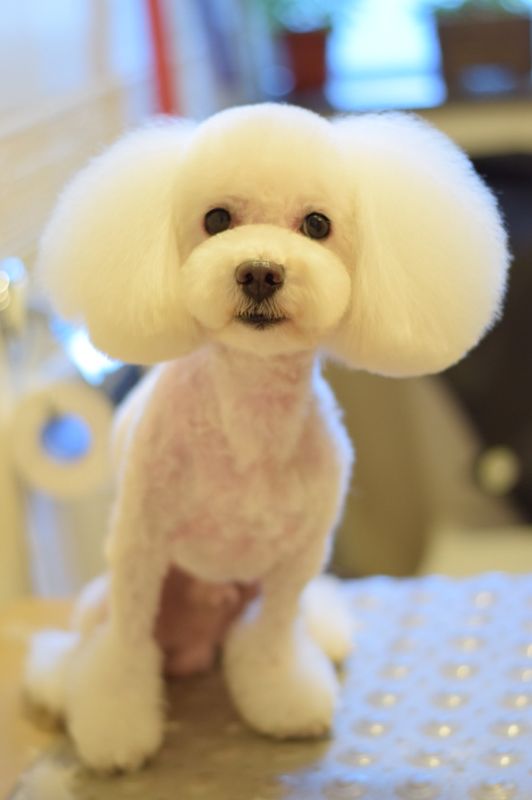The image features a small white poodle sitting on a table with a blue-tinted tablecloth. The dog’s grooming style draws focus, having been shaved around its neck, chest, body, and most of its legs, revealing some pink skin beneath its short white fur. In contrast, the dog’s head, ears, snout, and feet showcase enduring fluffiness, with its ears resembling cotton balls and its paws enveloped in longer fur. The dog has a round face, characterized by cleanly visible black eyes, snout, and mouth, set against its predominantly white, fluffy coat. The background suggests an indoor setting, possibly a home, with out-of-focus elements including a window and some objects. The portrait-oriented photograph, centered on the dog's face, captures a realistic and detailed representation of the freshly groomed poodle staring directly at the viewer.